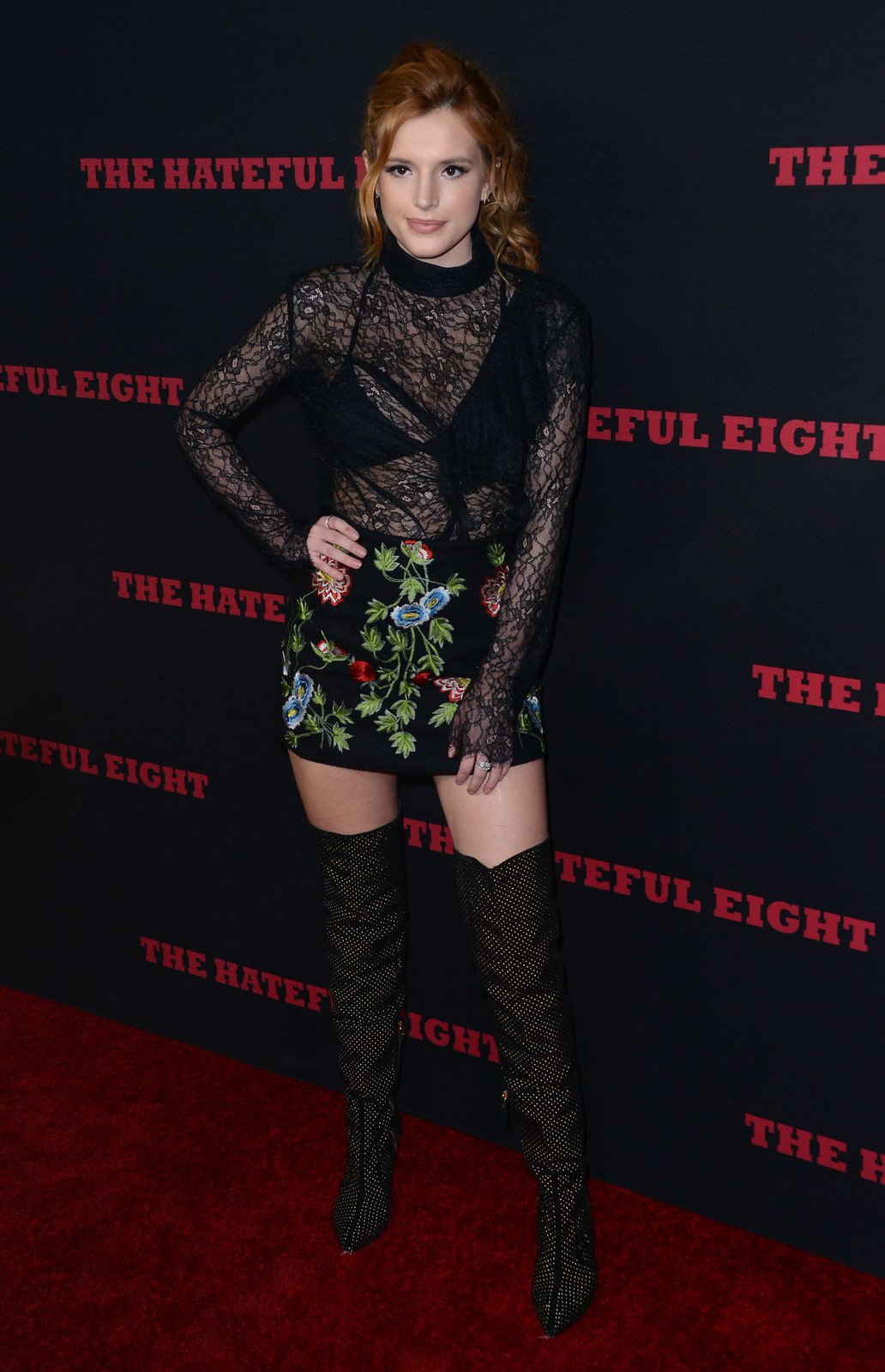In the image, a woman with fiery red hair is posing confidently on the red carpet for the movie "The Hateful Eight." Behind her, the black backdrop features the movie's title in bold red lettering. She exudes style in her striking outfit: over-the-knee black boots with a hint of white, a black miniskirt adorned with a green vine and leaves, and a lace top revealing a black bra underneath. With one hand on her hip and the other held in front of her left leg, she radiates elegance and poise. The red carpet she stands on is a darker shade, almost reminiscent of blood, reflecting the film's intense themes. Her smile and self-assured stance make her a captivating presence against the thematic backdrop.